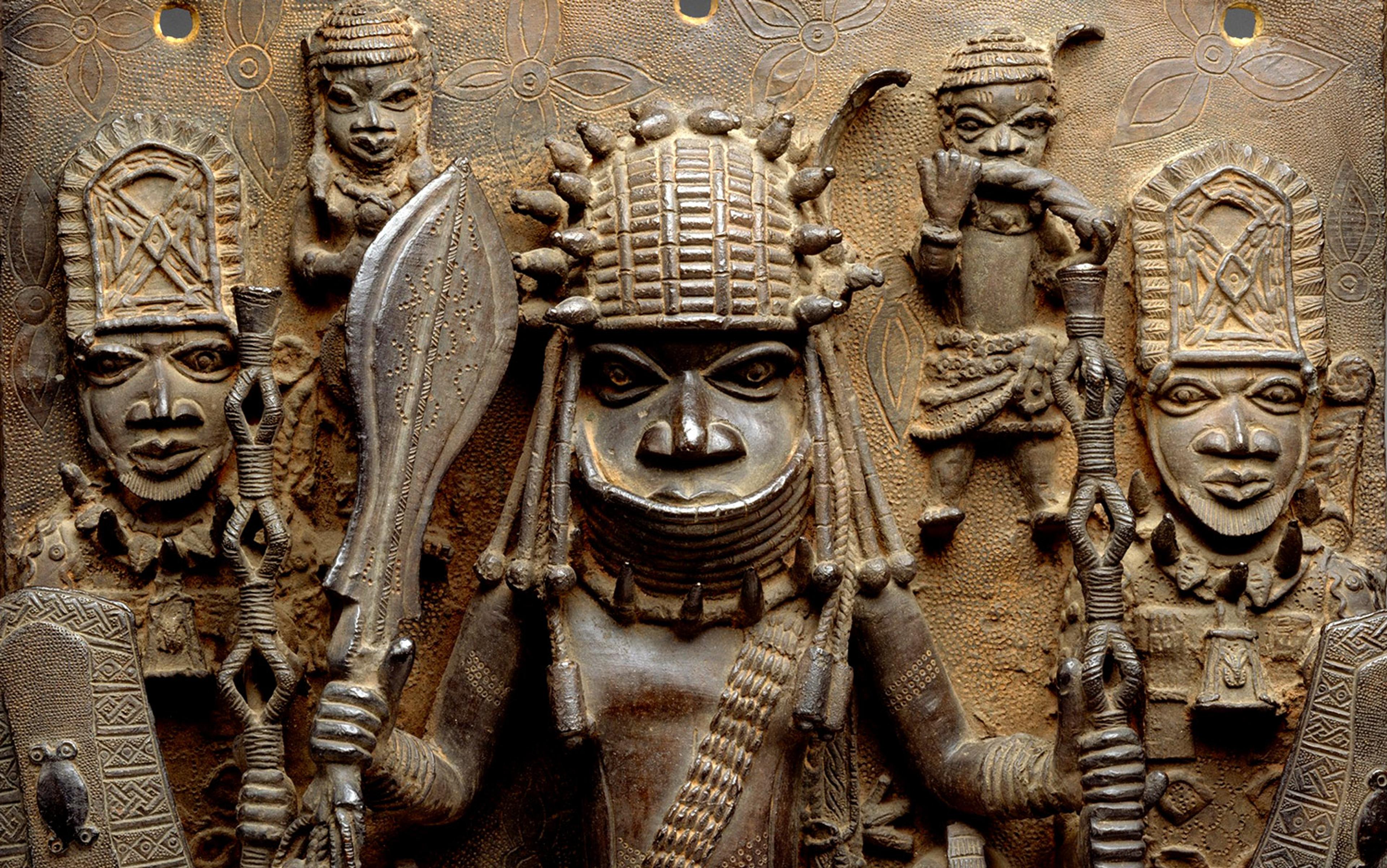The photograph features a detailed bas-relief carving, likely crafted from cast iron, showcasing five stylized African warrior figures. Each figure is adorned with primitive headdresses and simple attire, characteristic of traditional tribal aesthetics. The central figure, the most prominent, bears a sash across their chest and holds a weapon, possibly a sword, indicative of a leader or a person of significant stature. Flanked behind this main figure are two smaller figures, possibly representing children or lesser warriors. The remaining figures also brandish traditional African weapons such as spears and shields, illustrated with a rounded and elongated design typical of primitive African cultures. The background of the carving is decorated with stamped floral patterns, adding depth and texture to the piece. The overall patina and intricate craftsmanship suggest that this historical relic was intended as a wall hanging, capturing the essence of African tribal art and storytelling.